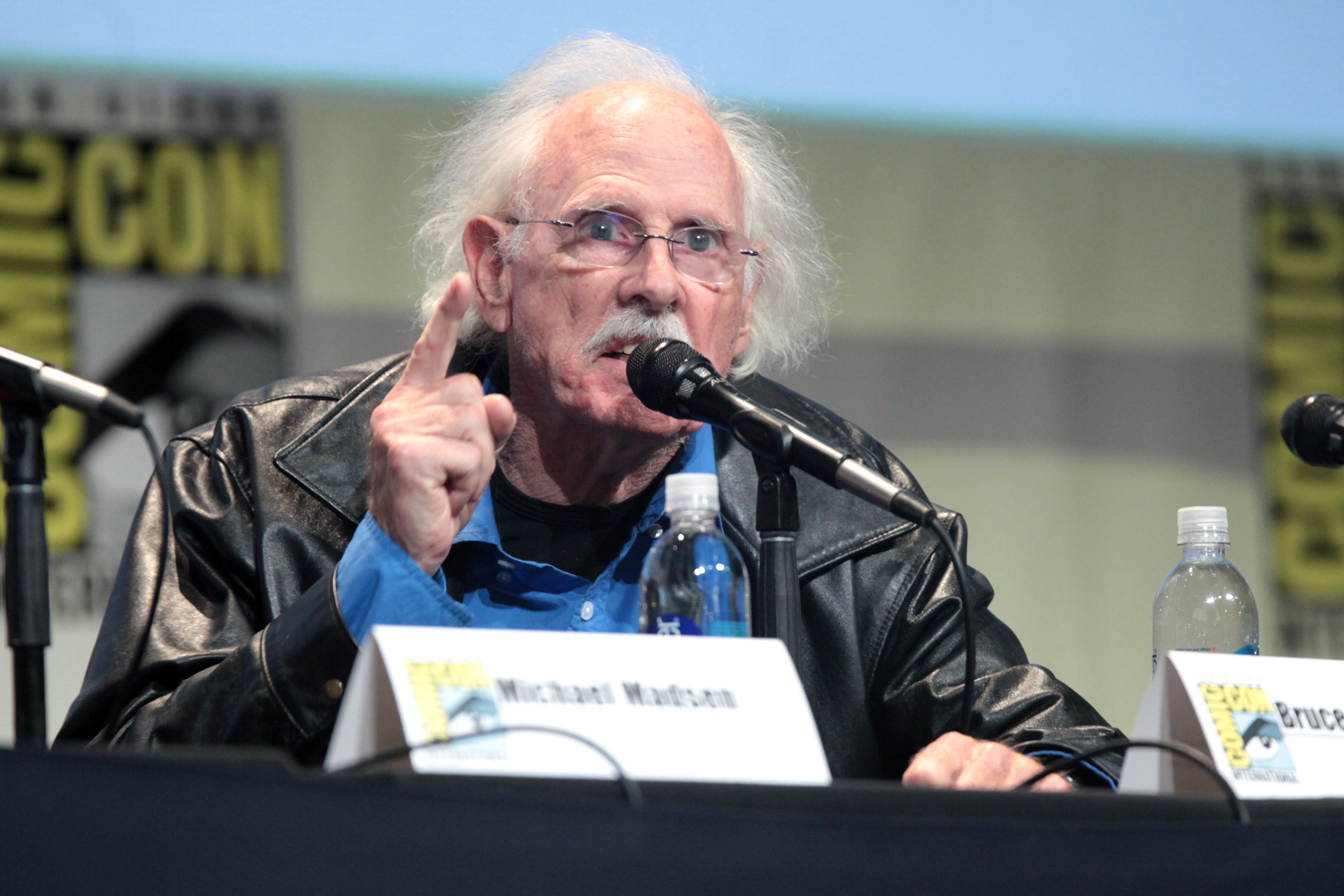In this detailed photo taken at Comic-Con, the focus is on Bruce Dern, an older gentleman with white hair, a white mustache, and rimless glasses. He is seated behind a black microphone on a black table, wearing a black leather jacket over a blue undershirt and an additional black shirt beneath. In front of him sits a water bottle and to his right, another water bottle shares the table. A name card displaying "Bruce" alongside the Comic-Con logo is partly visible to his right. The background features blurred Comic-Con logos, enhancing the event's setting. Bruce Dern is holding up his right hand with his index finger pointed upward, seemingly making an emphatic point during his speech.